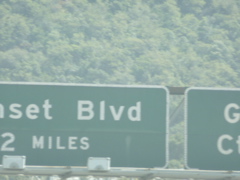This small, slightly foggy photograph captures a dense forest of dark green trees, tightly packed together with some lighter green foliage towards the top. The trees are so densely packed that no sky is visible, stretching from top to bottom and obscuring much of the background. Prominently featured in the image are two large, green overhead road signs attached to silver or gray metal arms that extend horizontally across the scene. The sign on the left, which reads "S-E-T Boulevard" and mentions a distance of "two miles", is partially cut off on the left edge. The sign on the right is mostly obscured, revealing only a "G" at the top and "C-I" at the bottom. Additionally, there appears to be a grayish platform along the bottom edge of the signs with possible lamps that might illuminate the signs at night.